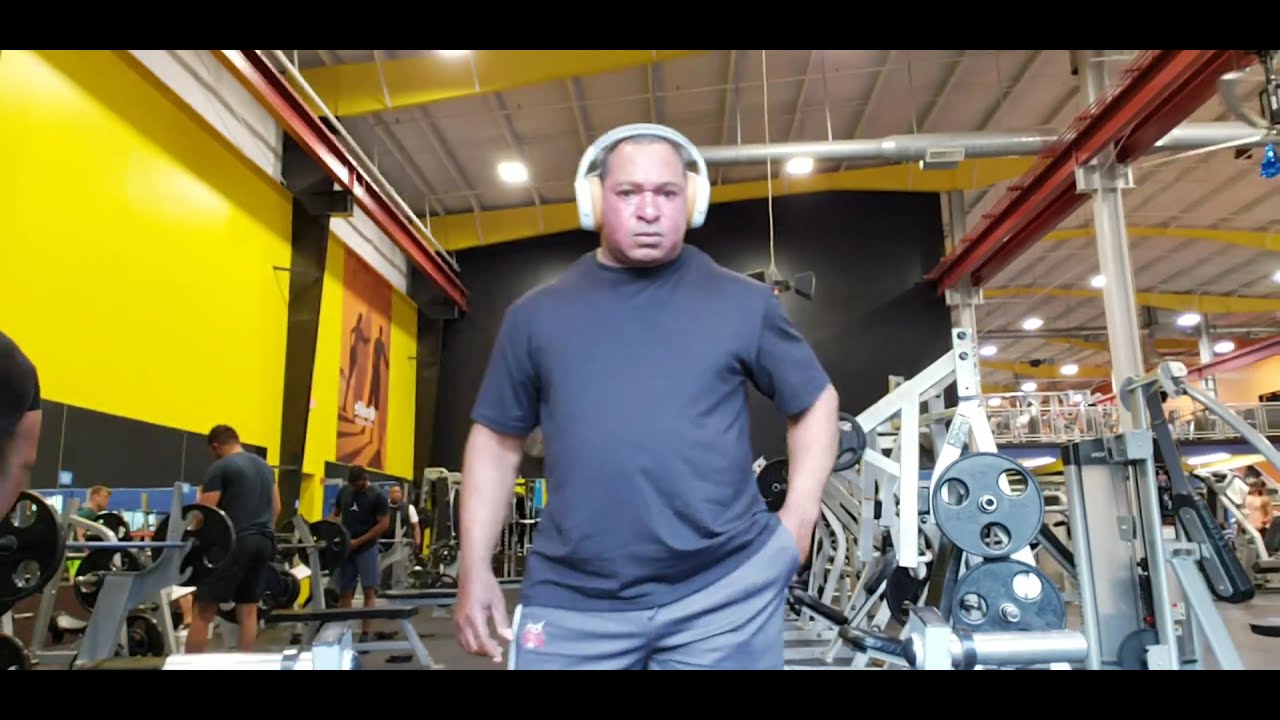The photograph captures a man in a large, warehouse-style gym, characterized by its high ceilings and spacious layout. The man, somewhat overweight, is wearing a gray shirt, gray shorts, and white headphones. He seems to be looking down at something with a worried expression. Surrounding him are numerous people engaged in various exercises, all dressed in athletic gear, adding to the bustling atmosphere of the gym. The gym features an assortment of weightlifting equipment and likely includes treadmills. The walls are predominantly bright yellow, with a contrasting black wall visible in the distance. There’s also a fitness poster on one of the yellow walls. Overhead lights hang far above, illuminating the entire space, which also houses a red crane-like structure supporting additional gym apparatus.